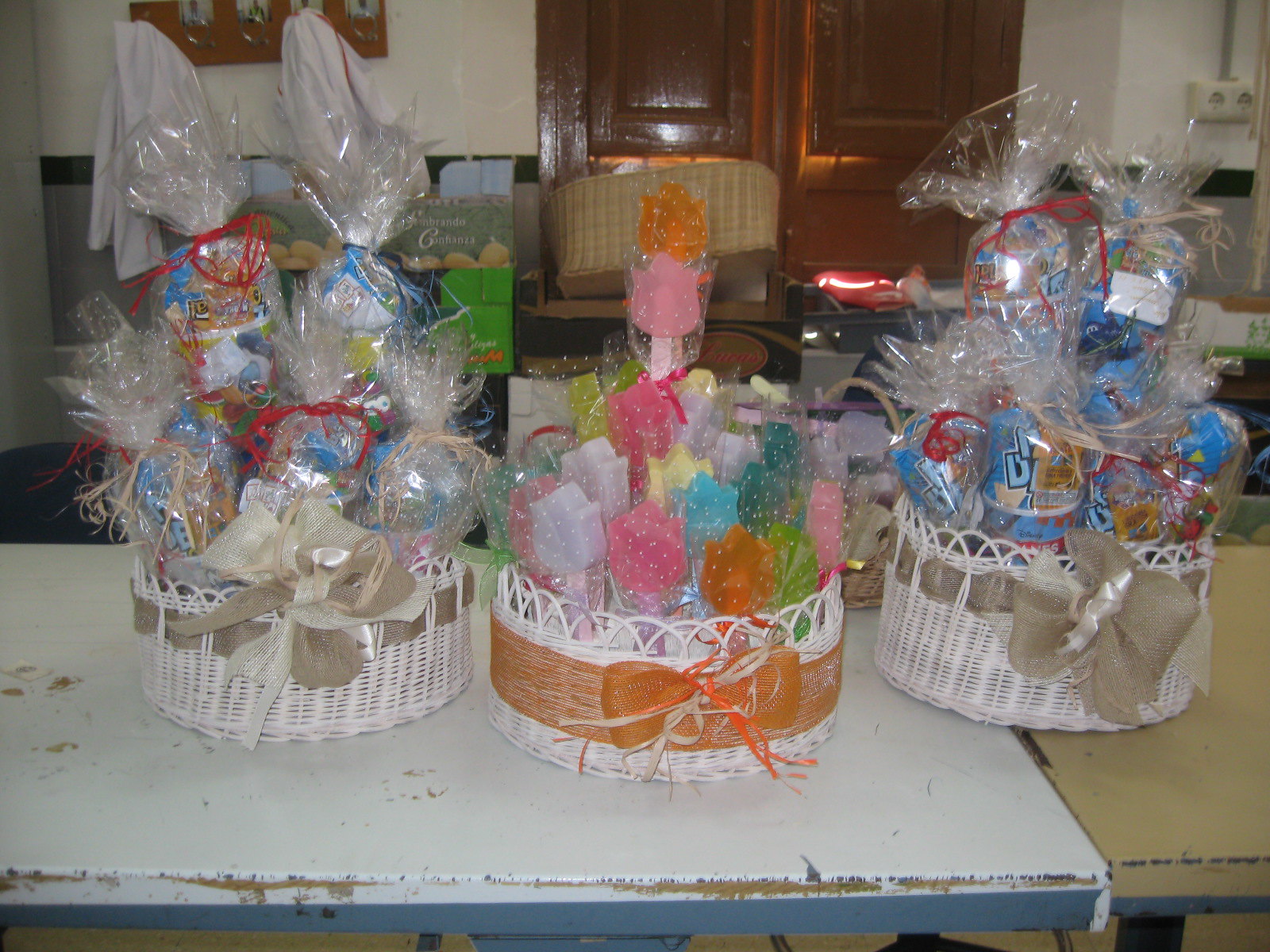This indoor photograph, possibly taken in a kitchen, features three white, woven gift baskets arranged on a table. The table consists of two sections pushed together—one being white and the other tan, both bordered in blue. The background includes a white wall and brown cabinets, with a woven basket adding to the cozy setting.

The two outer gift baskets are adorned with gray-brown bows, while the center one boasts a burnt orange bow. Inside the middle basket, there are various colorful items wrapped in plastic, showcasing hues of magenta, pink, orange, blue, and green; these items resemble lollipops or decorative soaps. The baskets on either side contain items primarily in blue and red, also wrapped in clear cellophane, which appear to be snacks or treats. Each basket is arranged meticulously, with the red and brown ribbons adding a touch of elegance.